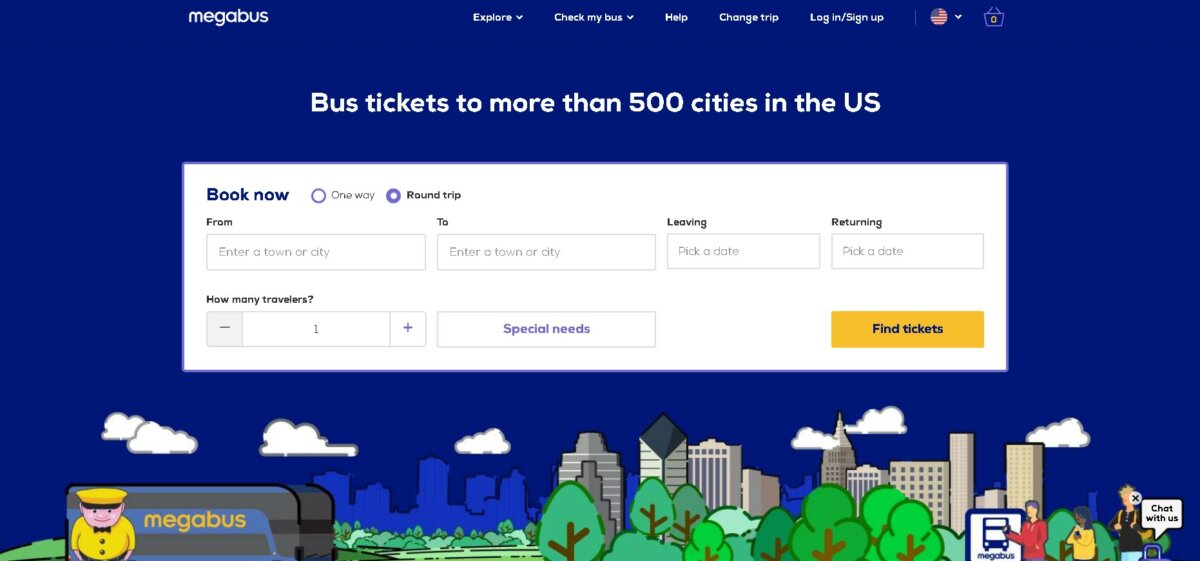Screenshot of Megabus Ticket Booking Page:

The image is a screenshot of the Megabus ticket booking page, prominently showcasing the user interface for purchasing tickets. The top section of the page features a navigation bar with options: "Megabus Explore", "Check My Bus", "Help", "Change Trip", "Log In", and "Sign Up", accompanied by an American flag icon and a shopping cart, all set against a blue background.

Below, a headline reads "Bus Tickets to More Than 500 Cities in the U.S." with a prompt to "Book Now". Users are given the option to book either a round trip or a one-way trip within a gray box. The booking form requires the user to fill in departure and arrival cities, select departure and return dates, specify the number of travelers, and indicate any special needs. An orange button labeled "Find Tickets" is situated at the bottom of the form for submitting the information.

The lower portion of the page is illustrated with whimsical drawings of office buildings, small people, bushes, trees, clouds, and a cheerful bus driver. The driver is dressed in yellow, and "Megabus" is emblazoned on the side of the bus he is driving. The entire scene combines functionality with playful design elements to create an engaging user experience.